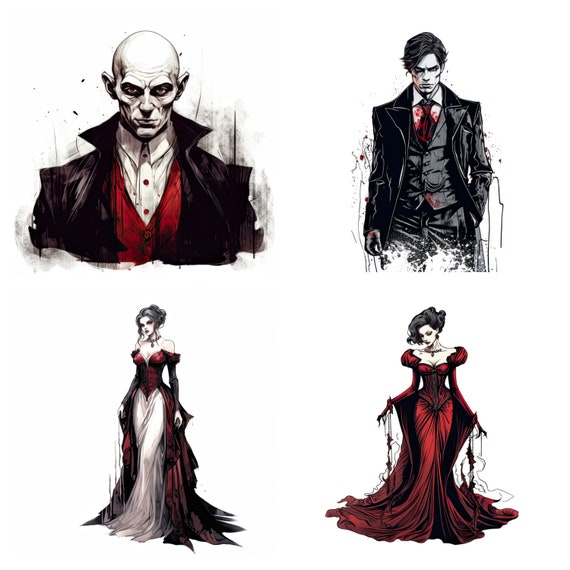This image contains a series of four meticulously detailed drawings, arranged with two men on the top row and two women on the bottom row, all unified by a vampire theme. Each character is distinct, but all share similar pale skin, formal attire in black, white, and red, and eerie features suggesting a vampiric nature. 

In the upper left corner, there is a bald male vampire with prominent ears and red eyes. His attire includes a traditional black jacket with a peaked collar, a red waistcoat, and a white button-up shirt with red buttons, enhancing his gothic appearance. To the right, another male vampire, younger and with dark, swept-over hair, is depicted in a black three-piece suit complete with a black tie and coat. His intense expression and blood-splattered shirt add to his menacing presence.

On the lower left, a female vampire is elegantly dressed in a fitted red and white dress that hugs her body before flowing outward. Her grayish-black hair and red gem jewelry complement her pale complexion. Lastly, the lower right drawing features another female vampire with black hair, clad in an elaborate scarlet dress that cascades onto the floor. Her crimson attire and matching jewelry, paired with her pale skin, make her look particularly regal and ethereal. 

Together, these drawings present a cohesive yet individualistic portrayal of well-dressed vampires, each embodying both elegance and horror.